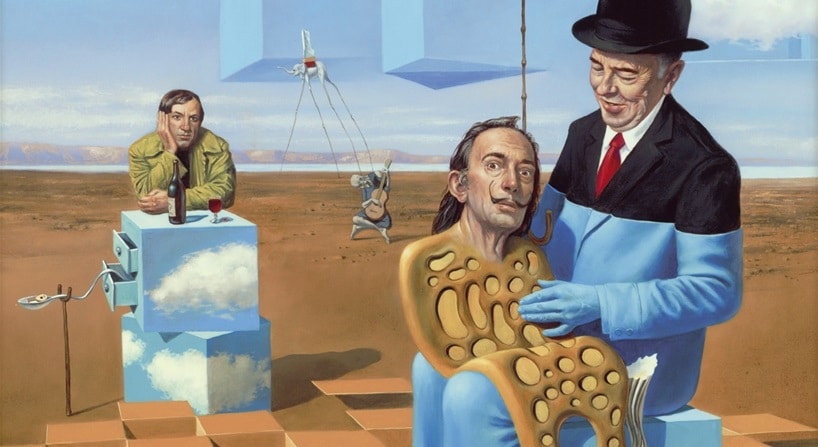The image is a horizontally aligned rectangular abstract art piece set in a desert-like area. On the right side, a man adorned in a suit jacket, red tie, and white collared shirt, along with a black hat, stands prominently. His suit's bottom part is enveloped in all blue, contributing to the image's artistic nature. His hand rests on another man with long hair and a thin, curled mustache, who gazes directly at the observer. The front of this man is obscured by a peculiar gold-colored object. 

On the left side of the image, another man leans against a pair of stacked blocks painted with images of the sky. The drawers of these blocks are open, and the man rests his face on his palm, giving a bored demeanor. In front of him is a bottle and a glass filled with red liquid, likely wine.

In the background, an uncanny human figure plays an oversized guitar. Further into the background, a giant elephant with exceedingly long legs towers above, almost reaching the sky. The sky itself is dotted with geometric shapes and appears cloudy with varying shades of blue. The scene unfolds on a barren, desert-like landscape, creating a surreal and dreamlike atmosphere.